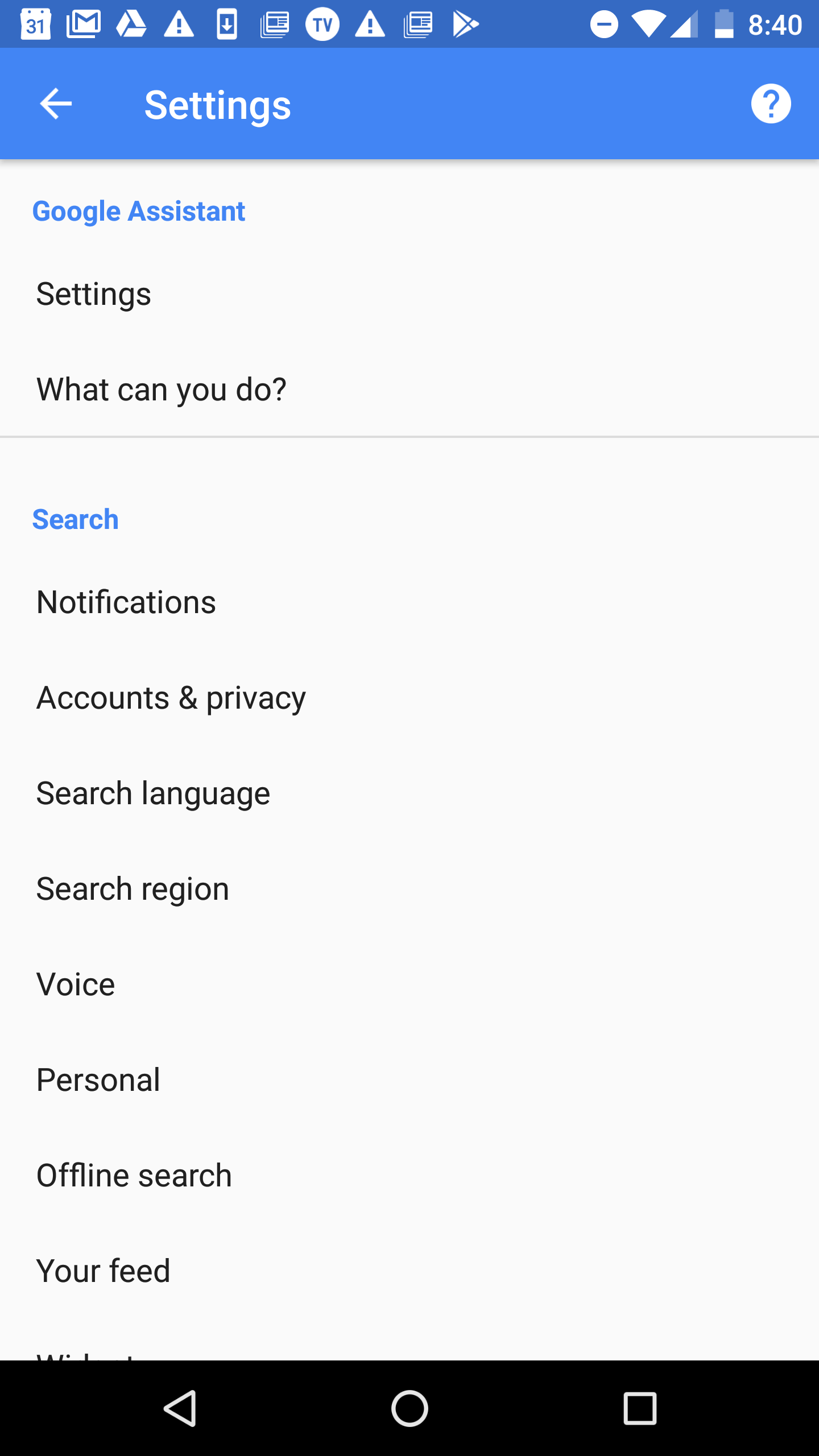The image depicts the interface of the Google Assistant app on an Android device. The top portion of the screen shows the device's status indicators and notifications. Starting from the top left, there are icons for a calendar set to the 31st, a Gmail notification, a Google Drive alert, and a warning symbol represented by a triangle with an exclamation mark. Additionally, there are notifications for a download in progress, a news organization, a TV icon with a circle, another warning triangle, more news alerts, and a Google Play Store notification. 

In the top right corner, the status indicators reveal that cellular data is turned off, Wi-Fi is enabled, the battery is at approximately 30%, and the current time is 8:40 AM. 

Below these status indicators, the screen displays the settings menu of the Google Assistant app. The options listed include "Settings" at the very top, followed by "Google Assistant," "Settings" (likely a sub-category), "What can you do," "Search," "Notifications," "Accounts and Privacy," "Search Language," "Search Region," "Voice," "Personal," "Offline Search," and "Your Feed." The final option partially visible at the bottom indicates that the settings menu is scrollable for more options.